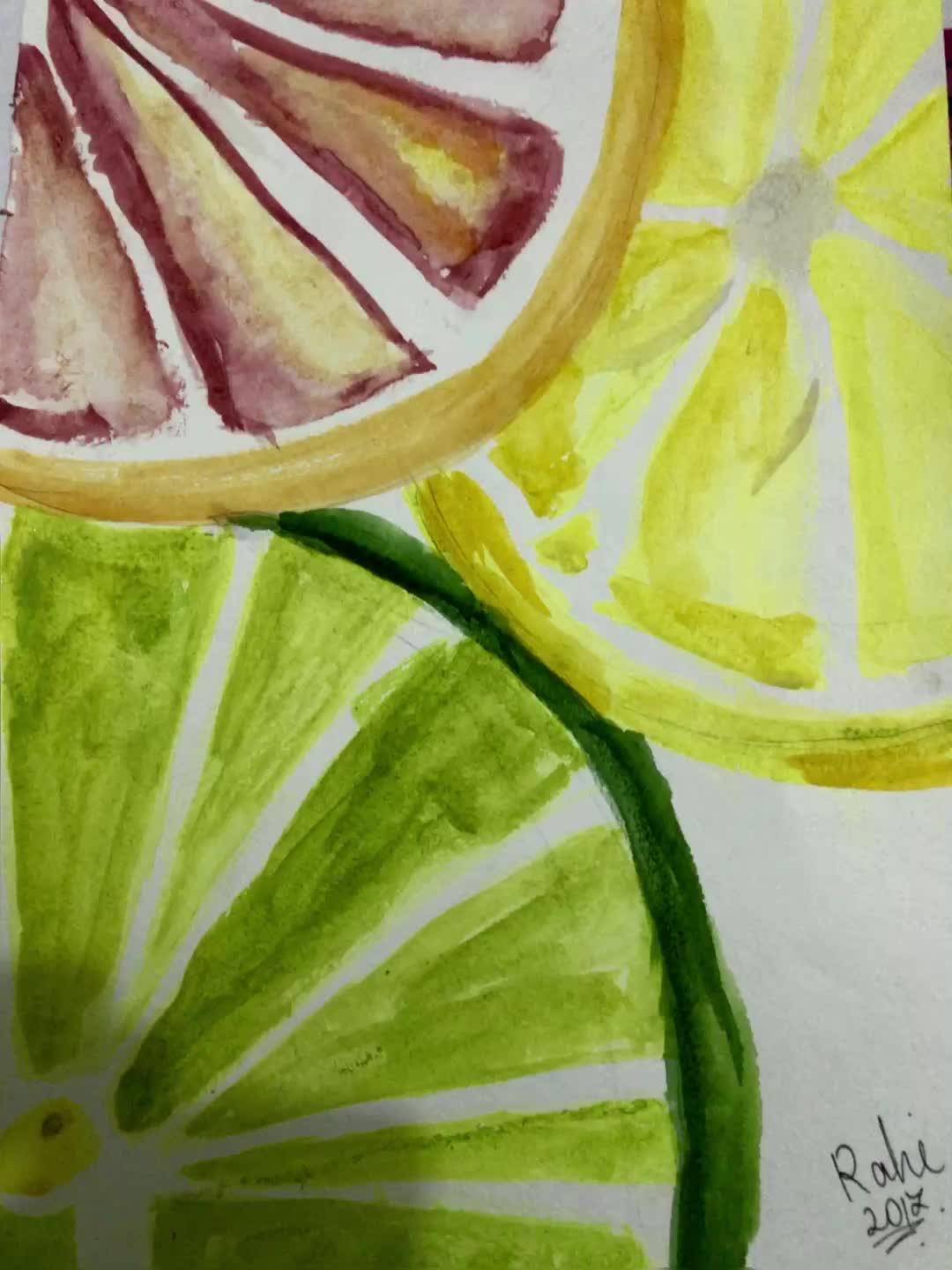This photograph showcases a vivid, Impressionist painting of citrus fruit sections on a white background. The painting features three overlapping fruit slices: a lime in the lower left, depicted with various shades of green and a dark green peel; a lemon in the upper right, displaying bright yellows and a pale rind; and a pink grapefruit (or possibly a blood orange) in the upper left, with dark pink to brick red segments and a dark yellow to orange peel. The colors are vivid and stylized, with all slices detailed yet impressionistic, likely created with acrylic paints. The artwork is signed "R.A.H.I. Rahi 2012" in black ink in the lower right corner, with a squiggly line emphasizing the number seven in the date.